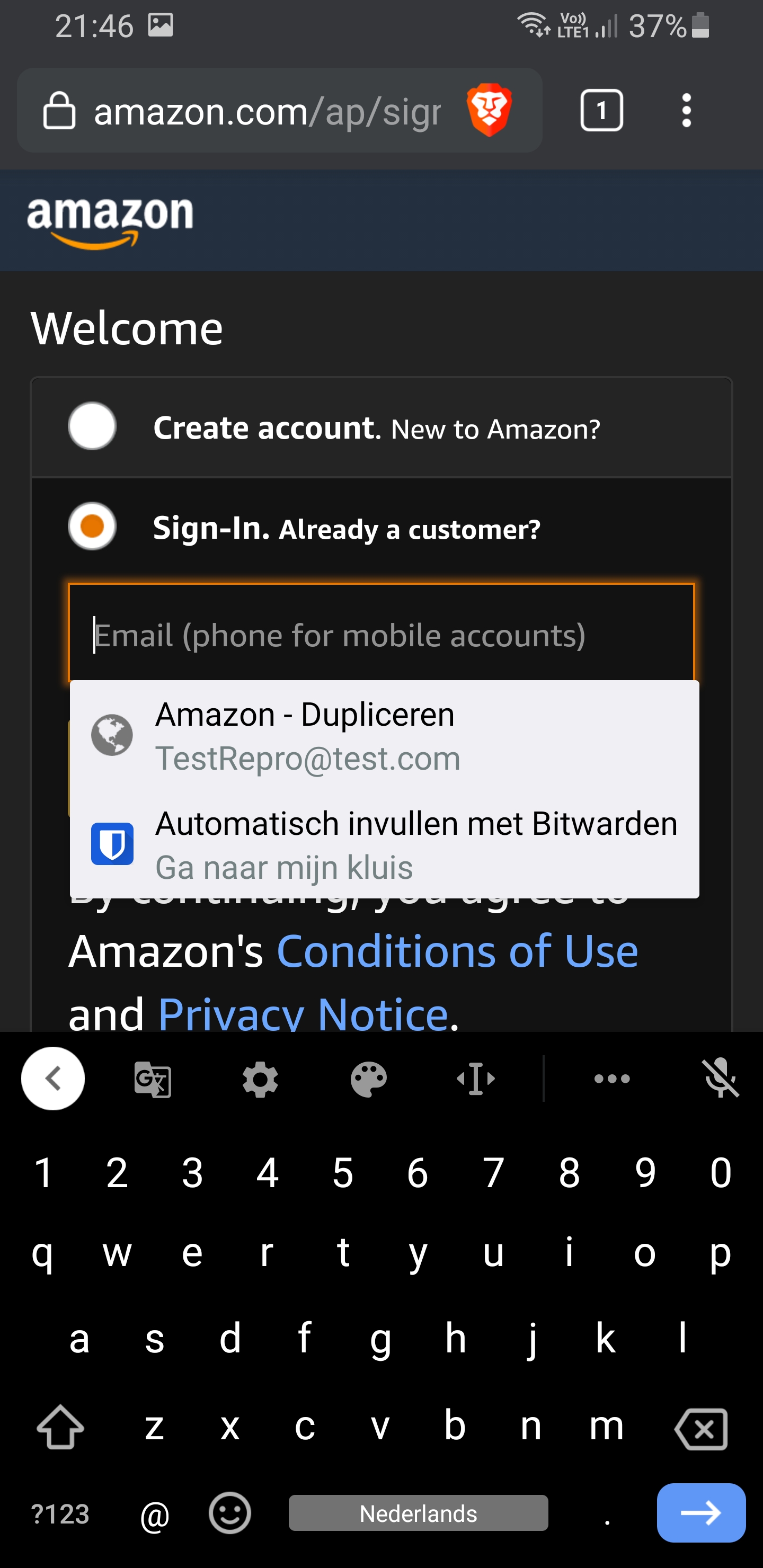A cell phone screenshot displays the Amazon sign-in page. At the top of the screen, a secure web address begins with a lock icon followed by "https://www.amazon.com/ap/signin". Adjacent to the address bar, a lion face icon and a tab indicator showing the number "1" are visible. To the right, a vertical three-dot menu icon is present. Below this upper section, a bluish bar features the Amazon logo in white font with an orange Amazon arrow beneath it. The background turns darker as the page welcomes the user with "Welcome" in white font. Beneath this greeting, options are provided: "Create your Amazon account," for new users, and "Sign-In," for existing customers. The "Sign-In" form is selected, with the cursor active in the email input field, showing a dropdown list of previously used email addresses.